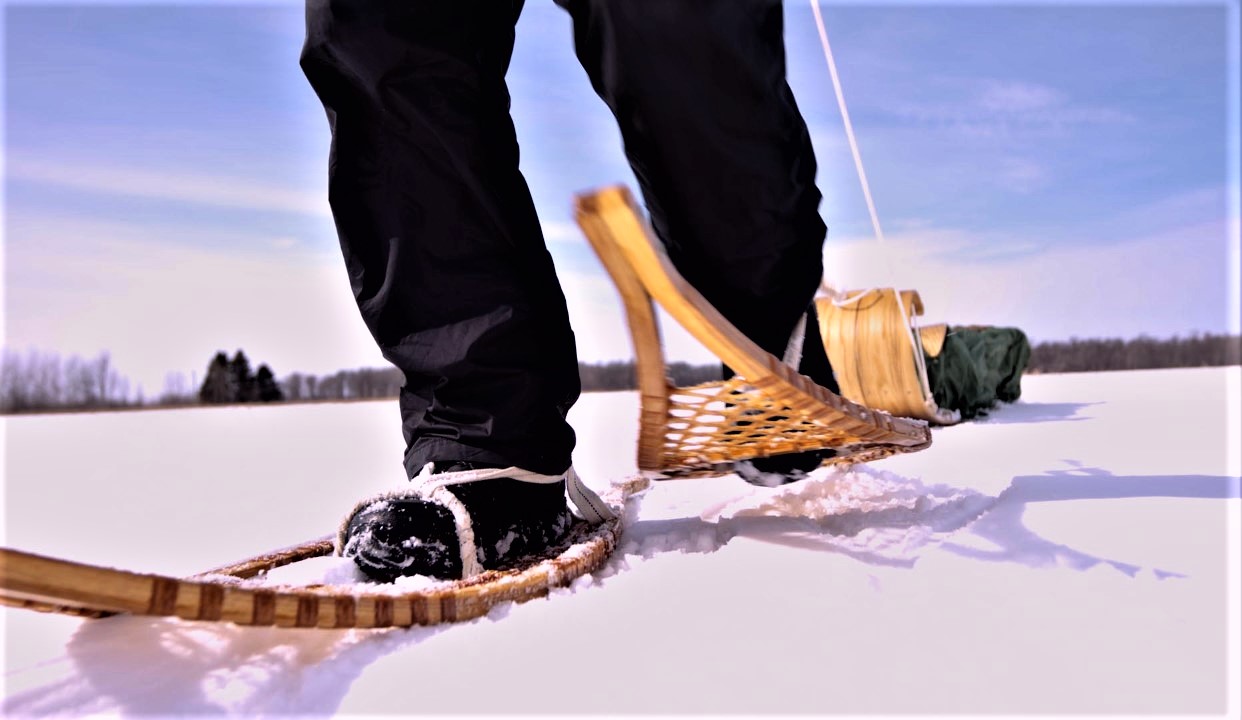In this close-up outdoor shot, a person dressed in black snow pants and black boots is seen from the knees down, walking through a snow-covered landscape in snowshoes. The snowshoes are made of light tan wood with traditional webbing, attached securely to their feet. One snowshoe is lifted mid-stride, indicating movement. The person is holding a thin white rope, pulling a wooden sled behind them. The sled, made of light brown wood, has a green blanket or cloth draped over it, concealing its contents. The scene is set on a flat, snowy expanse that could be a frozen lake bed, surrounded by a distant line of trees and a forest. A blue sky with wisps of white clouds stretches above, and a small mountainous structure and more trees are visible to the left.